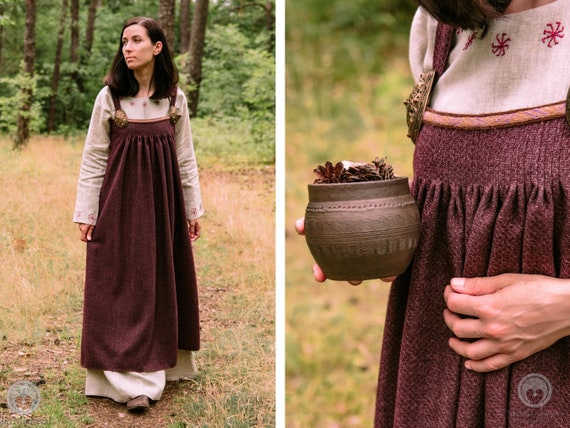The image consists of two vertically aligned photographs divided by a white line. On the left, a full-length portrait captures a woman with long brown hair standing in a small field. She is wearing an old-fashioned white cotton dress under a long brown apron dress, complemented by dark leather shoes. Surrounding her are lush green bushes and tall trees, adding a serene natural backdrop. The woman is looking to the left, giving a contemplative air to the scene.

The right side features a close-up of the same woman, focusing on her midsection. Her head is cropped out, but the details of her attire become more pronounced. She holds a small bronze pot by her waist, which is filled with pine cones. The apron dress's texture and the white dress beneath it are more visible in this frame, with the background blurred, continuing the woodland surroundings. 

Overall, the paired images present a juxtaposition of wide and detailed views, highlighting both the woman's antique attire and her interaction with nature.